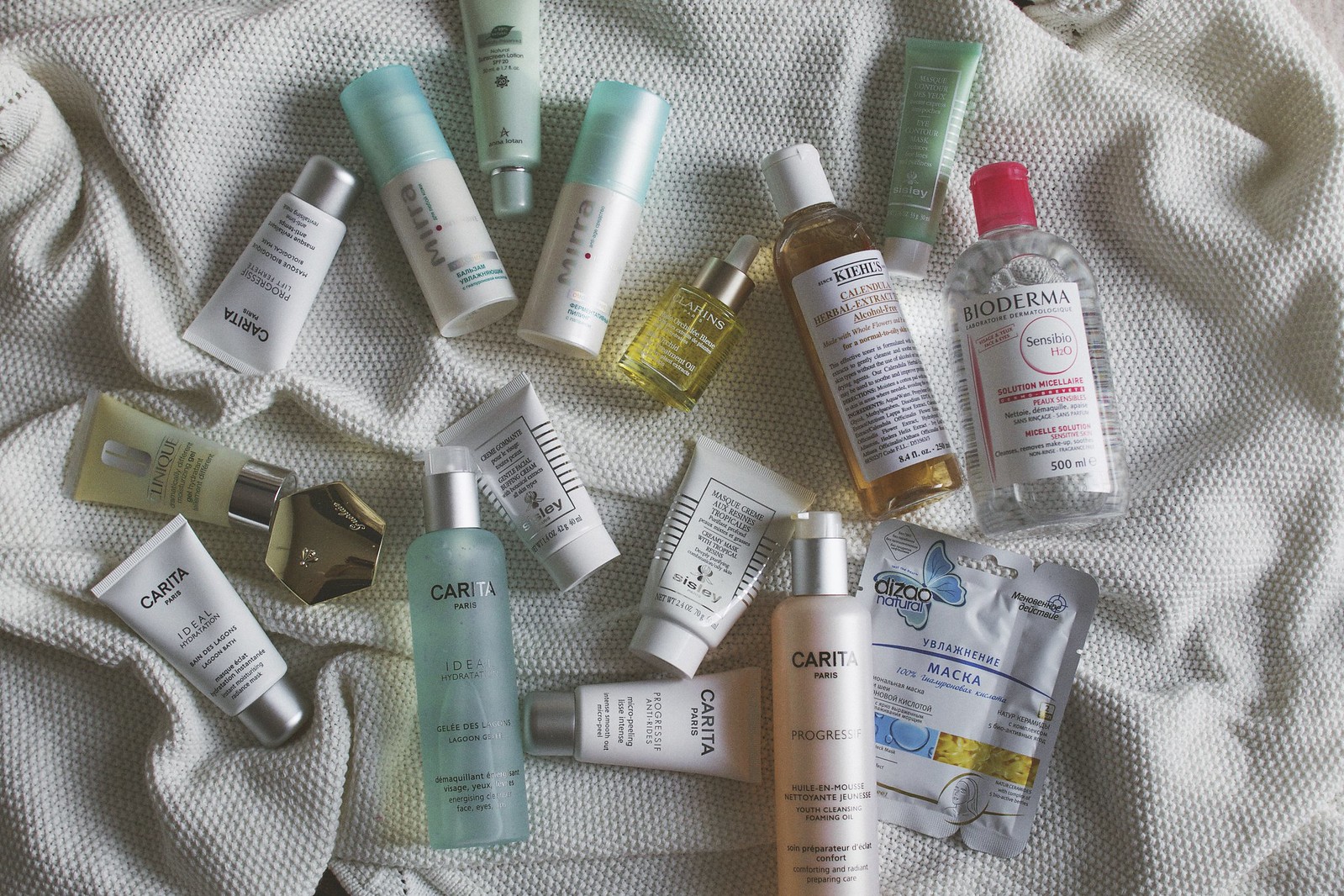This detailed photograph showcases a piece of crumpled white fabric adorned with shadows and folds primarily on the left side, creating intriguing gray areas. Strewn across the fabric are approximately 15 assorted bottles and tubes of facial and skincare products, seemingly haphazardly scattered as if a bag of makeup and lotion samples had been tipped over. Among the various items, one prominently features the brand name "CARITA" in Paris on a white label. While examining further, it becomes evident that the tubes all belong to the same manufacturer, Carita, whereas the bottles vary in origin. The assortment includes bottles filled with amber liquid, solid white bottles, and even a seafoam green bottle, adding to the colorful confusion. Each item lies in a random orientation—diagonally, upside down, and horizontally—enhancing the chaotic feel of the arrangement, which appears as if it fell from the sky and landed on the fabric.